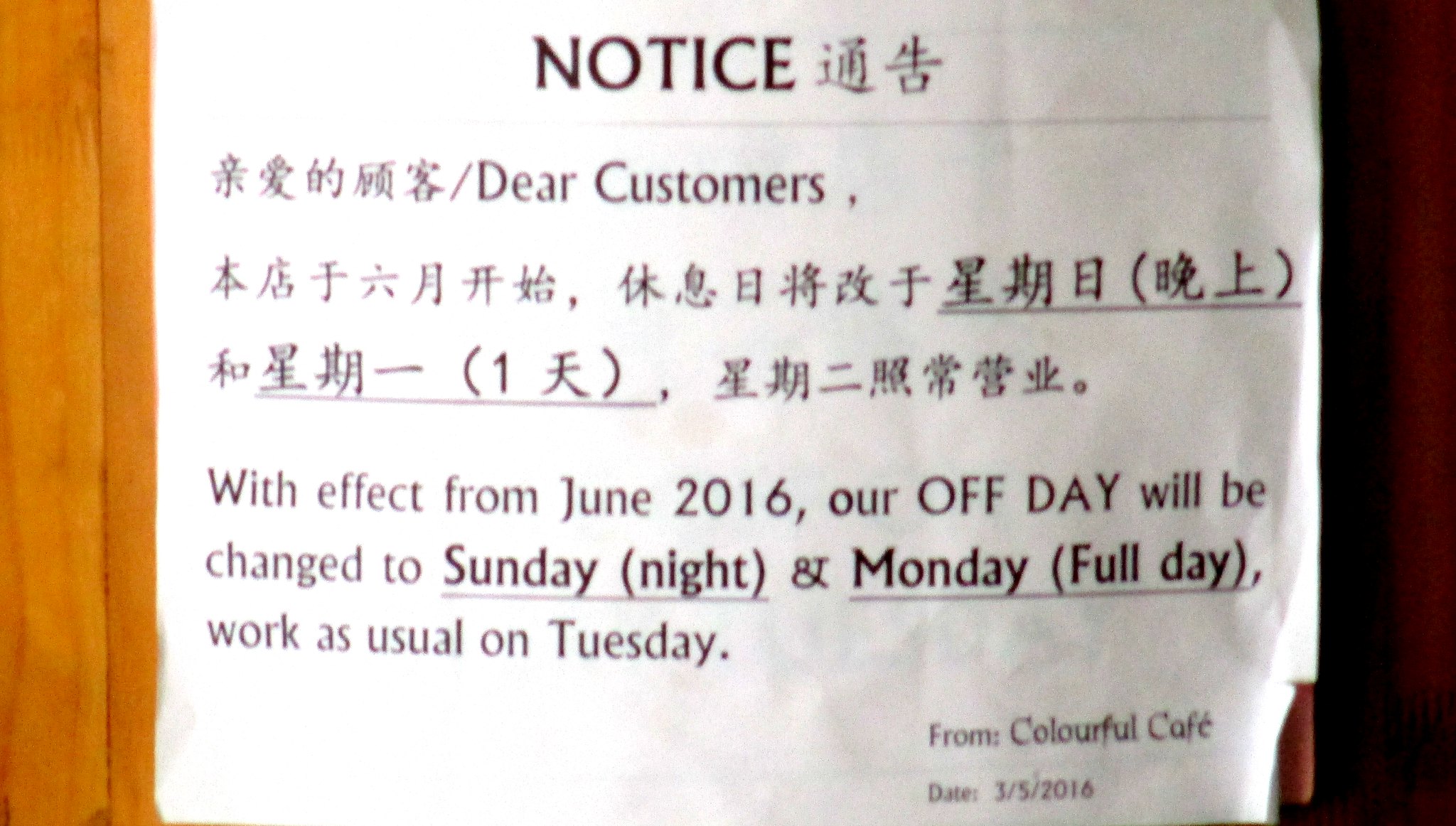This image captures a printed notice displayed against a backdrop of brown wooden paneling. The notice is printed on a white, rectangular piece of paper. At the top, it prominently displays the word "NOTICE" with a series of Japanese or Chinese characters beside it. Beneath, the text switches between the foreign script and English, addressed to "Dear Customers." 

The English part of the notice reads: "With effect from June 2016, our off day will be changed to Sunday (night) and Monday (full day). Work as usual on Tuesday." This message is signed off by "Colorful Cafe" and dated 3-5-2016. 

The paper additionally features a vertical yellow strip on its left side. The setting suggests this notice is posted indoors, possibly near a door, hallway, or passageway visible at the right edge of the frame. The detailed language and multi-lingual format indicate it is meant to inform customers about a change in business hours, specifying the new schedule for the cafe’s off days.